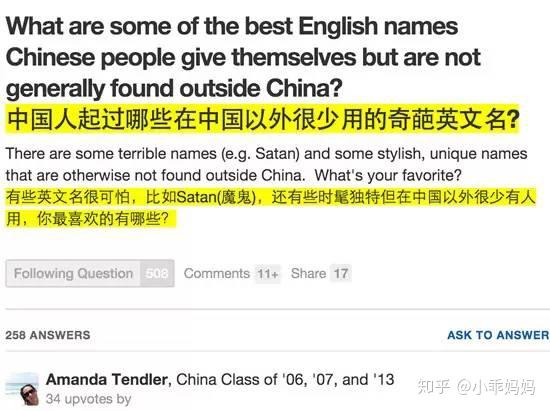A detailed caption for the image described:

"This image is a screenshot, likely from a computer, showcasing a discussion post with a white background and predominantly black text. The content revolves around the topic 'What are some of the best English names Chinese people give themselves, but are not generally found outside China?' featured prominently in bold at the top. Beneath this heading is a line of Chinese text, highlighted in yellow, presumably translating the question. The post continues with a smaller English text stating, 'There are some terrible names, e.g. Satan, and some stylish, unique names that are otherwise not found outside China. What's your favorite?' Additional Chinese text follows, also highlighted in yellow, ending with a question mark.

Below the text, there is an interactive box with options like 'Follow Question,' 'Comment,' and 'Share.' The post mentions '258 answers' to the question posed. The first response is from Amanda Tendler, indicated as having connections to China during the years 2006, 2007, and 2013. Her profile includes a small picture on the left side featuring a woman with dark hair and sunglasses. An excerpt of her response is visible, showing '34 upvotes by' before it gets cut off, leaving the remaining text unreadable."